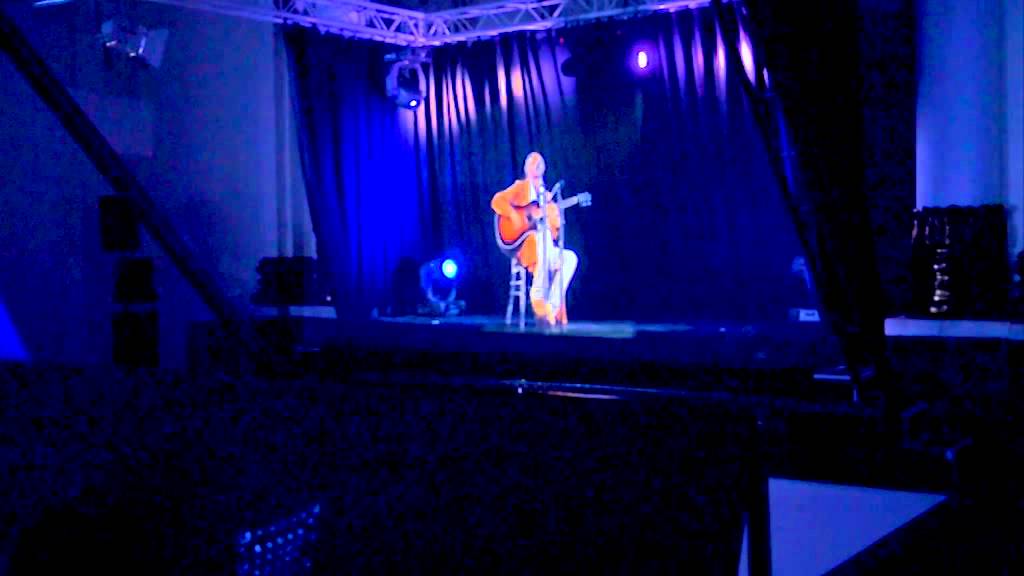The image captures an intimate concert scene in a small, dimly lit venue. Positioned in the audience, the view focuses on a lone male performer seated on a stool on a compact stage. A rich, deep blue and purple hue illuminates the stage, complemented by a spotlight that highlights the artist. He is dressed in an orange jacket, with a white shirt underneath, light-colored pants, and orange shoes. The performer holds an acoustic guitar, distinctively designed with a brown body and black border, and sings into a microphone. The stage backdrop features dark curtains that reflect the colored lights, intensifying the moody atmosphere. Although the audience is not clearly visible due to the darkness, the setting suggests an intimate performance, possibly in genres like blues or folk music. The image is somewhat blurry, rendering the performer's facial features indistinct.